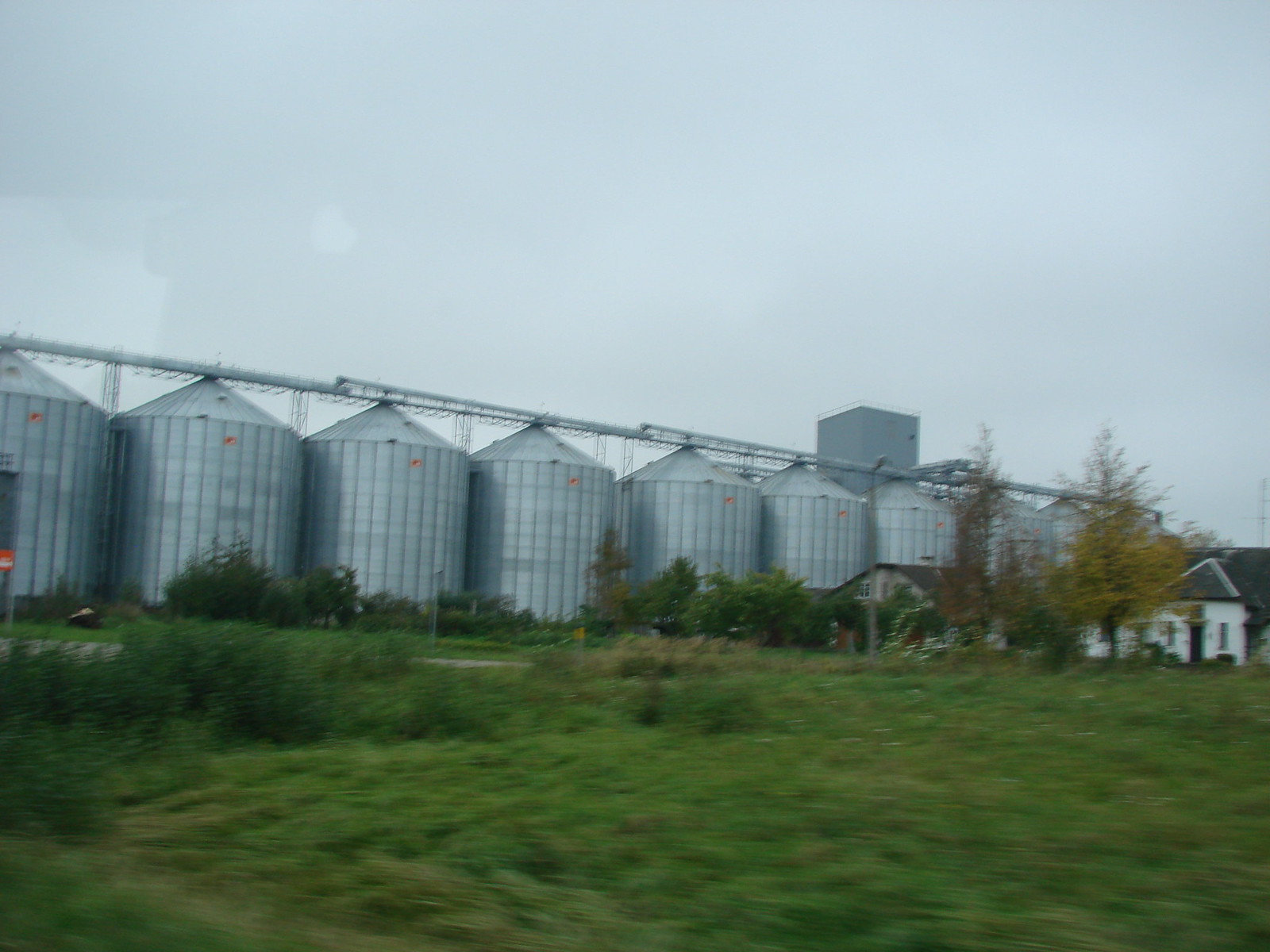The image features a row of about ten cylindrical grain silos, each topped with a flattened cone and interconnected by a network of slender metal bars or grates. The silos stretch from the left side of the image, where they appear closer and larger, to the right side where they diminish in size and become partially obscured by a couple of trees. The base of the silos is surrounded by green, tall, and somewhat windblown grass, occasionally sun-scorched in patches.

Adjacent to the row of silos are two buildings: a low brown building and a white building. The brown building has a reddish colored roof, and the white building, situated further to the right, has a brown roof. Between the buildings and the silos, there are several trees, with two notable ones featuring amber and orange leaves, respectively. The overall landscape suggests a farm-like setting with a mix of industrial and residential elements nestled together.